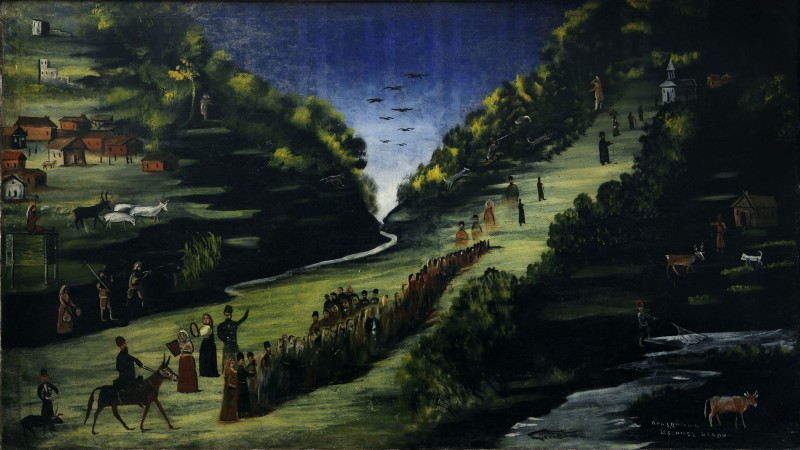This detailed artwork, possibly an oil or watercolor painting, portrays a vibrant countryside scene filled with diverse elements. The landscape features lush green hills and a grassy valley, interspersed with a small stream flowing through the terrain. In the middle of the painting, a road or path runs, lined shoulder-to-shoulder with a line of people. Various livestock, including cows and possibly goats, roam the grass, contributing to the bucolic ambiance.

The top portion of the artwork showcases a blue sky gradually fading to white as it meets the horizon, dotted with black birds flying in a curved formation. Green trees punctuate the hillside, and scattered throughout are small cottages and houses, adding a quaint charm. In the upper right-hand corner, a building, possibly a church, stands tall, and at the very top of the hill is a stark white church overseeing the serene landscape.

A fisherman, adorned with what seems to be a Russian headdress, tends to the stream, while a white dog and a deer stand nearby. Additionally, there are floating figures midway up the hill, surrounding which are men on horses and a donkey being ridden at the bottom left. The painting is rich with color, featuring hues of black, white, yellow, green, gray, blue, red, off-white, and tan. Finally, a small, intricate signature is scrawled at the bottom right-hand corner beneath a cow, adding a finishing touch to this enchanting rural scene.